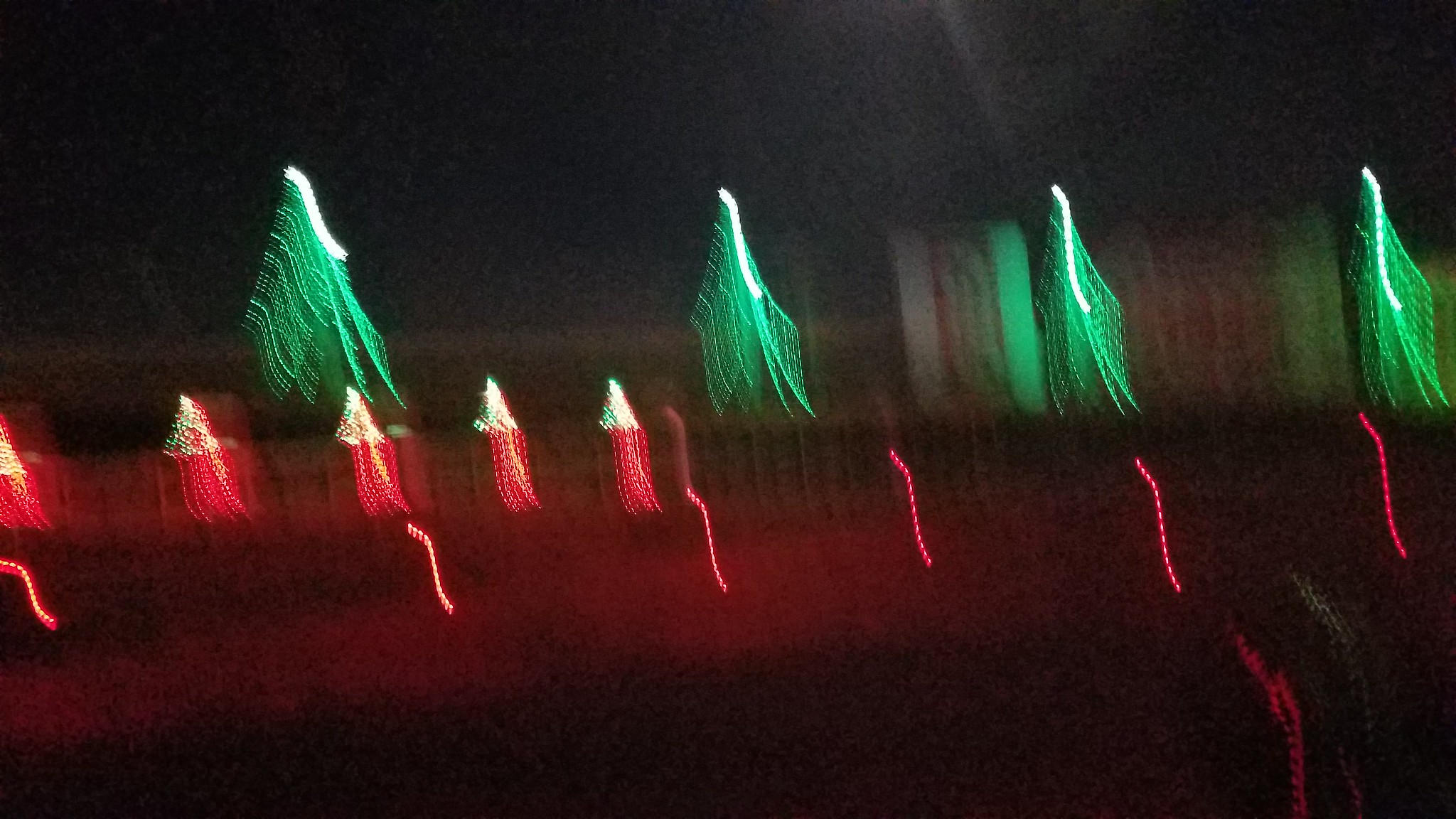This photograph captures a festive, albeit blurry, Christmas scene adorned with an array of colorful lights. The centerpiece is a group of green Christmas lights arranged meticulously into the shape of a traditional Christmas tree. These illuminated trees are placed on a raised platform, and behind them, one can spot an additional four or five similar Christmas tree light decorations, adding depth to the scene. A step down from these green lights reveals another row of decorations featuring red lights capped with white tops, resembling holiday stockings or stocking stuffers, with about five prominently displayed. Descending yet another step down, the front row showcases vibrant candy cane lights, characterized by their distinctive red and white glow, which frame the entire display of green Christmas trees and red stocking decorations, completing this cheerful holiday tableau.